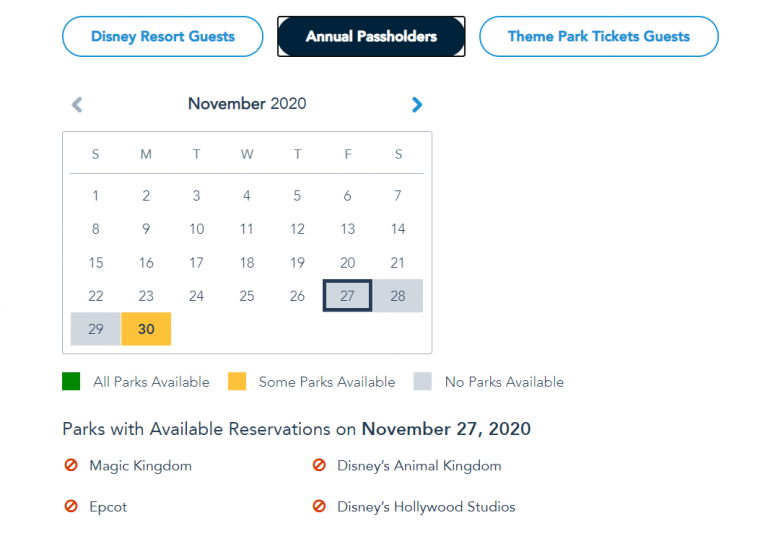The screenshot depicts a reservation calendar from Disneyland Resorts for the month of November 2020. At the top of the screenshot, there are three buttons: "Disneyland Resort Guests" in blue on the left, "Annual Pass Holders" in white on a black background in the center, and "Theme Park Ticket Guests" in blue on the right with a white background. Below these headers, the calendar prominently displays the month "November 2020."

A black box highlights the date Friday, November 27th, and the dates November 27th, 28th, and 29th are shaded in gray, indicating that no parks are available on these days. November 30th is marked with a yellow box, signifying that some parks are available.

Beneath the calendar, a legend explains the color codes used: a green box means "All parks available," a yellow box means "Some parks available," and a gray box means "No parks available." Additionally, the section titled "Parks with available reservations on November 27th, 2020," lists four categories: Magic Kingdom, Epcot, Disney's Animal Kingdom, and Disney's Hollywood Studios. Each category is marked with a red circle and a diagonal bar, indicating that no reservations are available for any of these parks on that date.